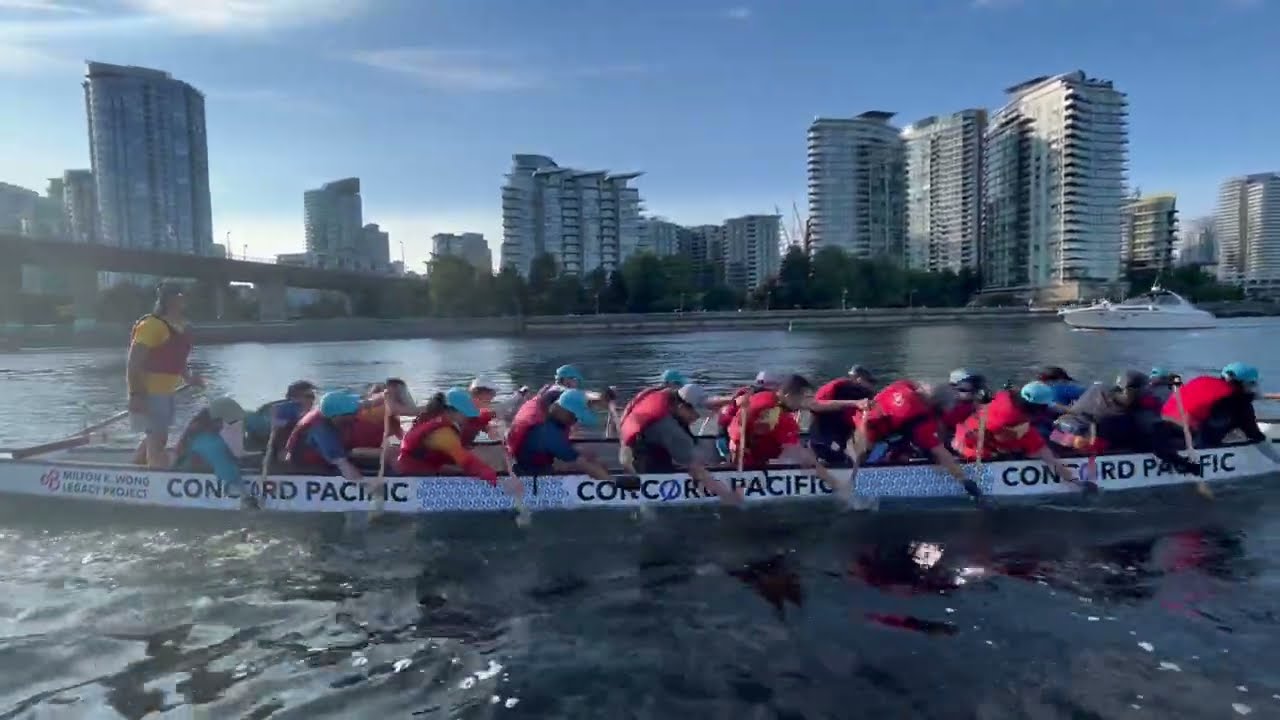The image depicts a vibrant scene of a sports team kayaking in orderly rows on a large kayak labeled "Concord Pacific." Comprised of 20 rowers clad in red life jackets and light blue hats, the team is further coordinated by one individual standing at the back. The backdrop boasts a picturesque cityscape with tall skyscrapers and a bridge to the left, and it's complemented by a few scattered clouds in the clear blue sky. The water, appearing very clear in the foreground, stretches out to reveal a white yacht on the right side, near a roadway. Trees line the area between the water and the city skyline, adding a touch of greenery to the urban environment. Additionally, the kayak features the inscription "Milford Milton E. Wong Legacy Projects" on its left edge, further enriching the scene.